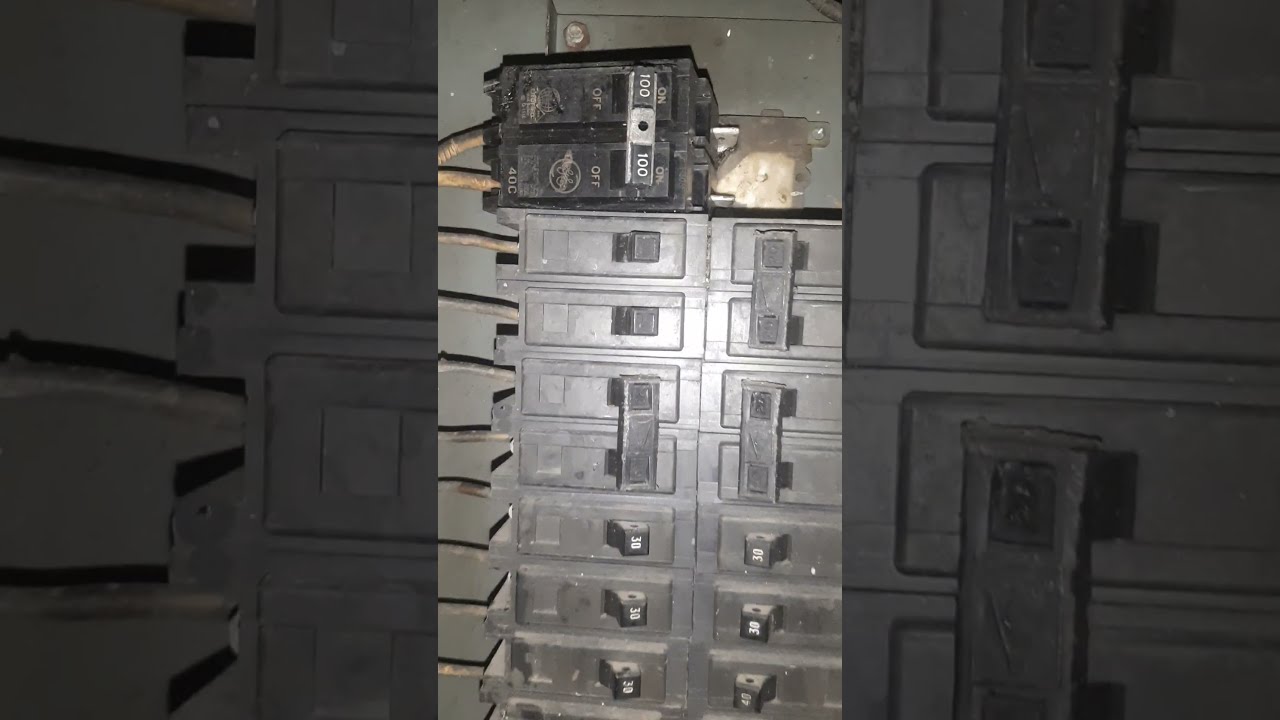This is a detailed portrait mode cell phone photograph of an electrical circuit breaker box. The central focus of the image is a gray metal panel housing multiple circuit breakers, flanked by darker, shadowy edges on either side. The top of the box features a black circuit breaker that appears to be loose and unattached from the panel. Among the cluster of breakers, some have black switches with white numbers, indicating various amperages such as 30 and 100. There are dirty yellow and gray wires protruding to the left of the breakers. The breaker switches are labeled with "ON" and "OFF" text, some in yellow. The image also reveals elements of wear and age, with dirty surfaces, old wires, exposed screws, and remnants of tape or glue. Notably, the General Electric (GE) symbol is visible on some of the breakers. The setting of the image is ambiguous, but it could plausibly be inside a garage or a home. The overall impression is of a close-up view of a well-used fuse box, with all its intricacies and signs of frequent use.